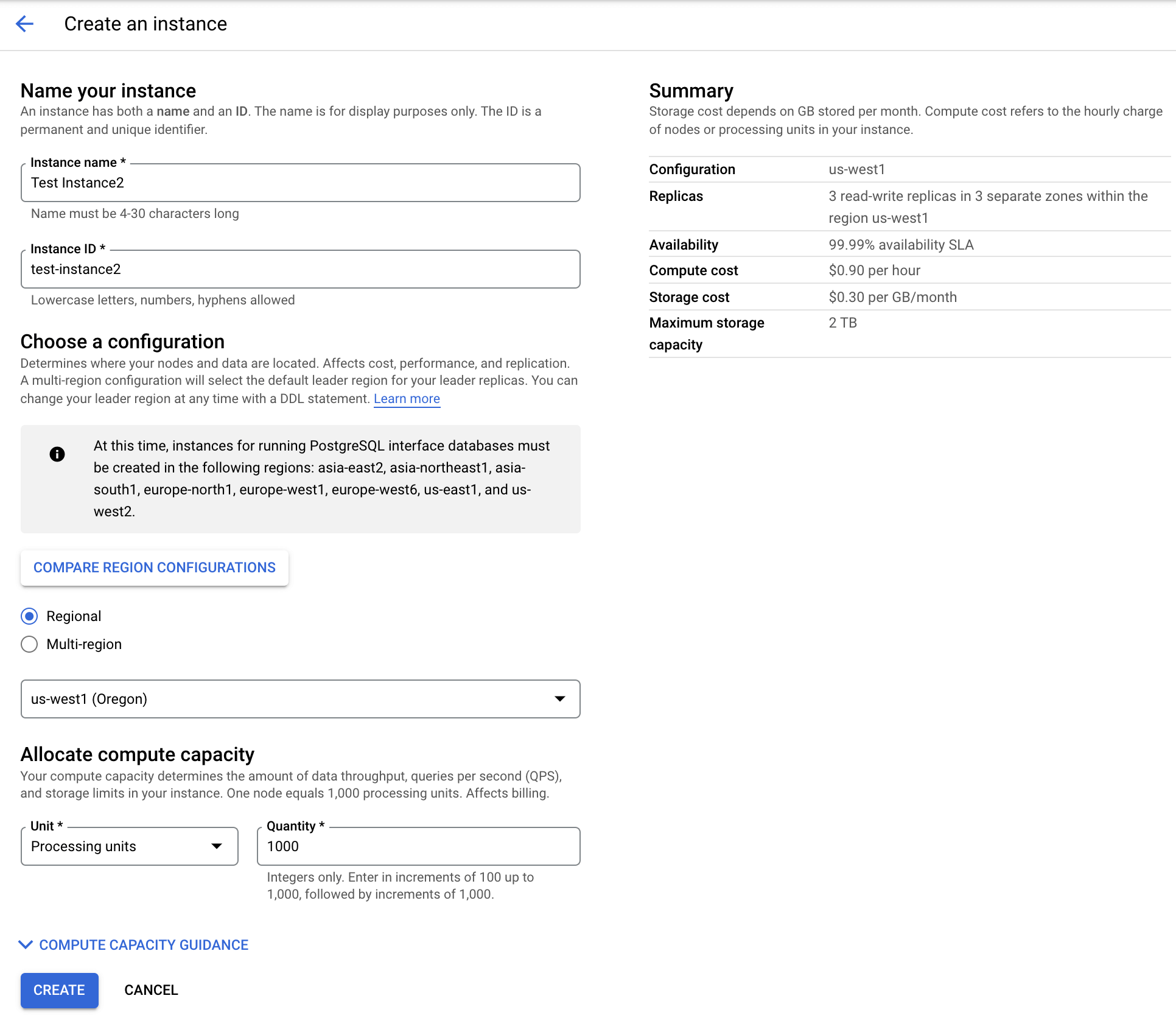A detailed image depicts a web page with a predominantly white background and predominantly black text. At the very top, a prominent heading reads "Create an Instance." Under this, the first entry box asks users to "Name Your Instance," with fields for "Instance Name" and "Instance ID."

The page is divided into two columns. The left column is densely populated with information, starting with a main heading, "Choose a Configuration," followed by options for "Regional" or "Multi-regional" configurations. Further down, another heading reads "Allocate Compute Capacity," with subheadings for "Compute Capacity Guidance."

The right column is about one-third full. Its main heading, "Summary," is followed by detailed data points such as "Configuration," "Replicas," "Availability," "Compute Cost," "Storage Cost," and "Maximum Storage Capacity."

At the very bottom, on the left-hand side, there are two interactive buttons. The left button is blue with white text reading "Create," while the adjacent button to the right is black with the text "Cancel."